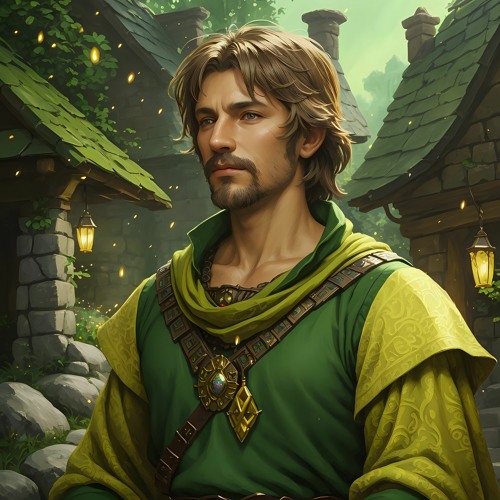This AI-generated cartoon image features a brown-haired man in his early thirties, dressed in detailed medieval attire. The man, who has a goatee, is clad in a green tunic adorned with gold-accented jewelry across his chest and around his neck. Over his tunic, he wears a dark green vest, while both the sleeves and collar of his outfit are a lighter shade of green. A noticeable feature is a strap or harness crossing his shoulders, possibly holding a central piece that looks like it has a stone. The backdrop includes a village of old stone and cobblestone buildings with slate or mossy wood shingle roofs. Lanterns hang on the walls to either side of him, illuminating the scene, which appears to be set at dusk. Additional elements in the background include several stone chimneys, columns, and smokestacks, with greenery peeking through. Fireflies float to the left and right of the man, adding a mystical touch to the evening setting.